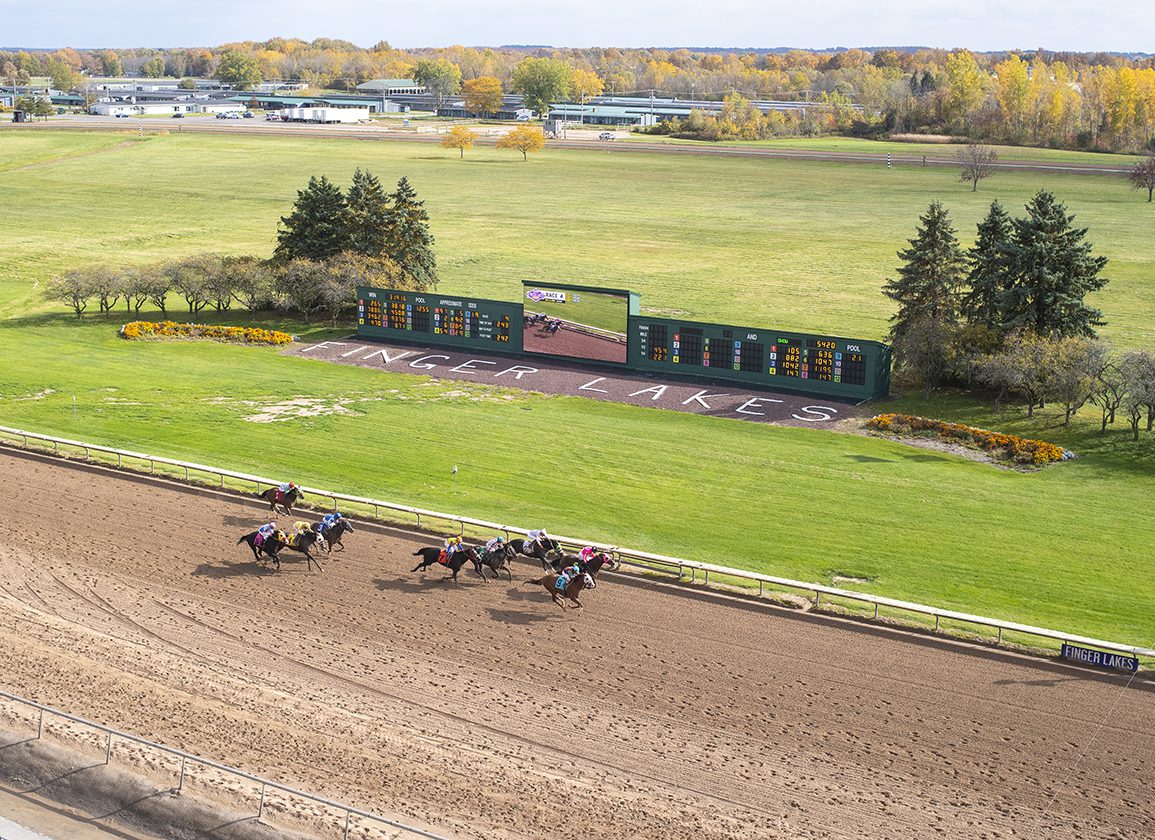The image captures an aerial view of the Finger Lakes horse racetrack, likely taken by a drone during an active race. At least nine horses with jockeys clad in colorful uniforms—pink, light blue, yellow, red, black, and white—are seen racing toward the finish line. The jockey in the aqua blue uniform is narrowly leading the pack, just ahead of one in a pink uniform. The dirt track is prominently featured, encircling a large grassy infield adorned with formal, decorative plantings of conifers, smaller trees, and flowering plants, which frame a significant video monitor and scoreboard. The inscription "Finger Lakes" is visible on the ground in front of the scoreboard, affirming the racetrack’s name. The ambiance suggests it's autumn, as evidenced by the trees with yellowing leaves. Beyond the racetrack, the landscape stretches to a complex of low buildings and rolling hills or mountains in the distant background, enhancing the natural beauty of the Finger Lakes region of New York.